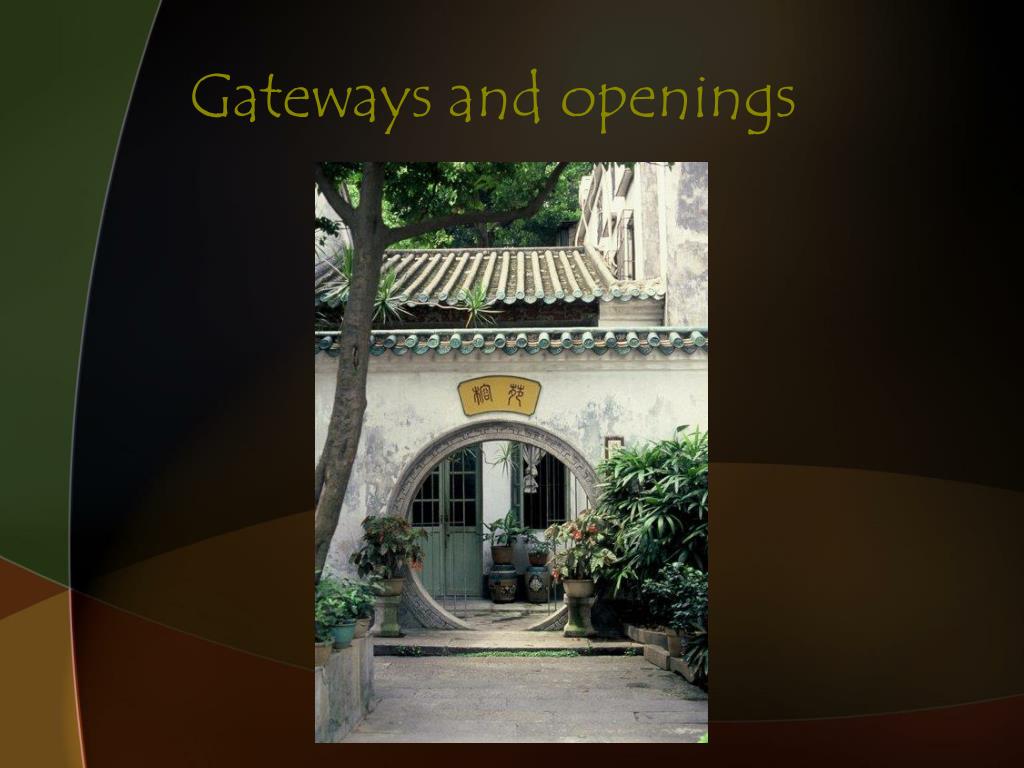The vertical, rectangular image features an old-style Asian building with a distinctive circular gateway. The building, primarily white with green and blue tinges from wear, appears to be constructed mostly of concrete. The circular entrance, almost a perfect circle with an incomplete bottom, is surrounded by a unique design and has a gold sign with Asian letters above it. To the left of the entrance, there is a tall tree, and more bushes and plants in potters are scattered across both sides, adding a lush greenery to the scene. The rooftop is adorned with some palm trees and bamboo, contributing to the serene atmosphere. This image, framed by a border with different shades of brown, olive green, dark red, and dark gold, features the words "gateways and openings" at the top in olive green. The blend of architectural elements and natural beauty gives it a unique and tranquil appeal, making it an inviting getaway.